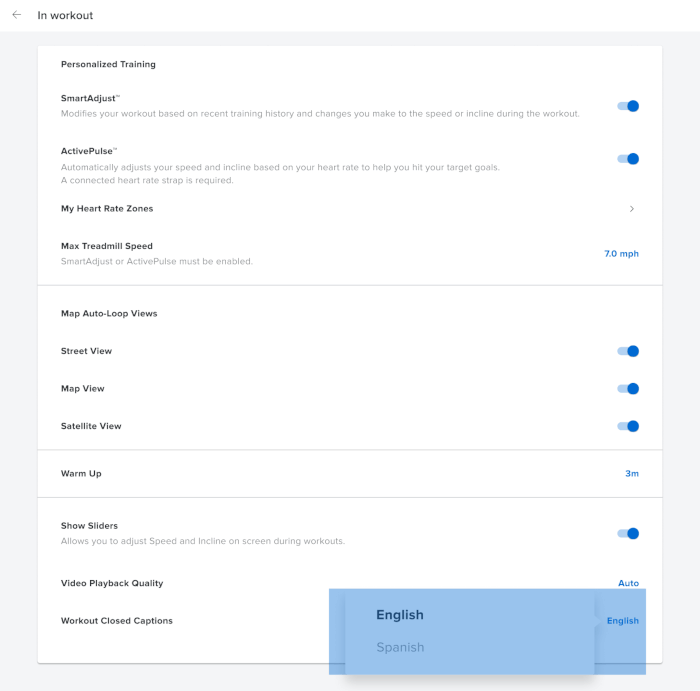The image features a white background with black text organized into various sections and adorned with icons and descriptors. At the very top, there's a single word aligned to the left, accompanied by a left-pointing arrow. Immediately to the right of this arrow, the text "in workout" is visible. Beneath this is a boxed area containing the phrases "personalized training," "smart adjust," "active pulse," and "my heart rate zones."

Next to these, towards the far-right side, the text "max treadmill speed" is prominently displayed with the number "7.0" beside it. Below this section, additional options are listed within boxes: "max auto loop views," "street view," "map view," and "satellite view."

Further down, another boxed area contains the word "warm up," next to which a right-pointing arrow denotes a duration of "3m" (3 meters). Below this, there are options for adjusting "show sliders," "video playback quality" (displaying "auto"), and "workout closed captions" (set to "English").

All sliders throughout the interface are active and illuminated. Finally, in the bottom right corner, there's a large blue rectangular button offering language options labeled "English" or "Spanish."